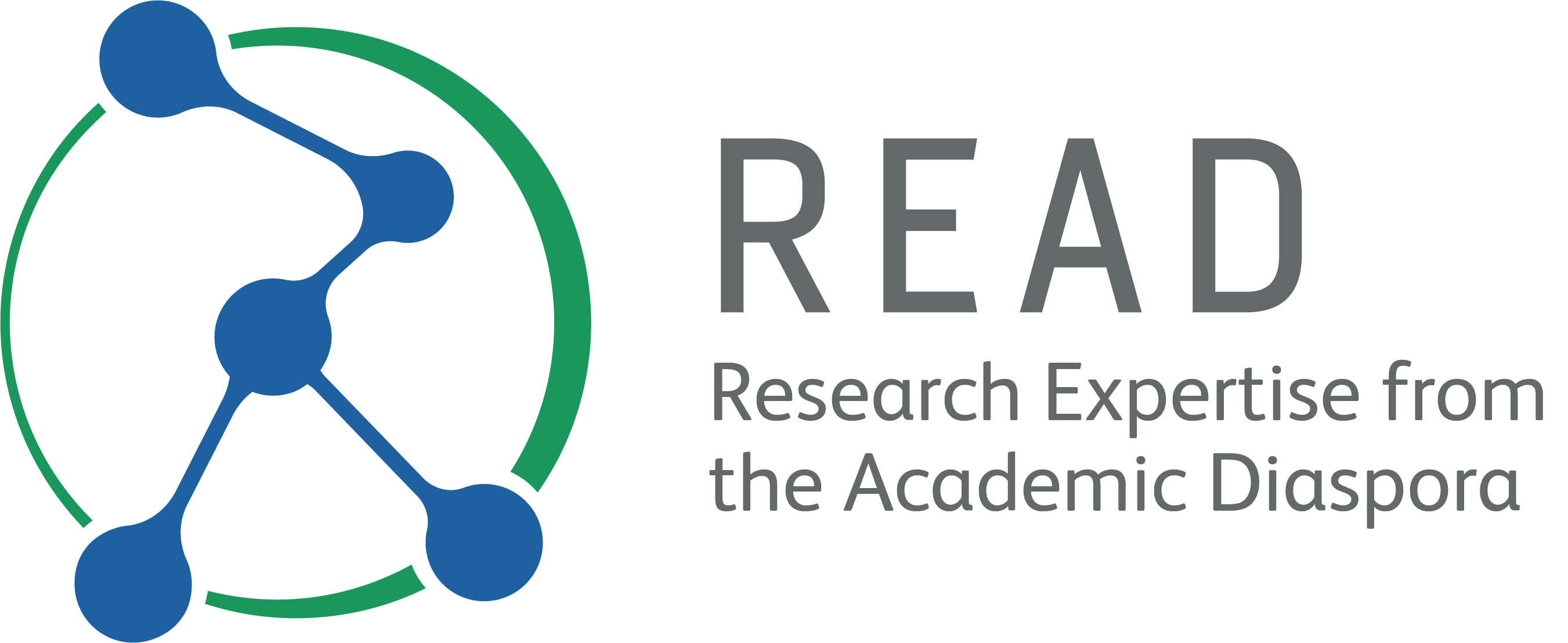The image features a prominently displayed logo on the left side, consisting of a large green circle. Within this green circle, there is a distinctive blue figure reminiscent of a Jax toy from childhood. This figure is composed of five solid blue circles connected by four thin blue lines, forming a unique pattern. To the right of this intricate logo, the word "READ" is prominently displayed in uppercase, gray letters. Directly below "READ," in smaller gray font, is the tagline "Research Expertise from the Academic Diaspora." The entire composition combines graphic elements with text to create a visually engaging design.